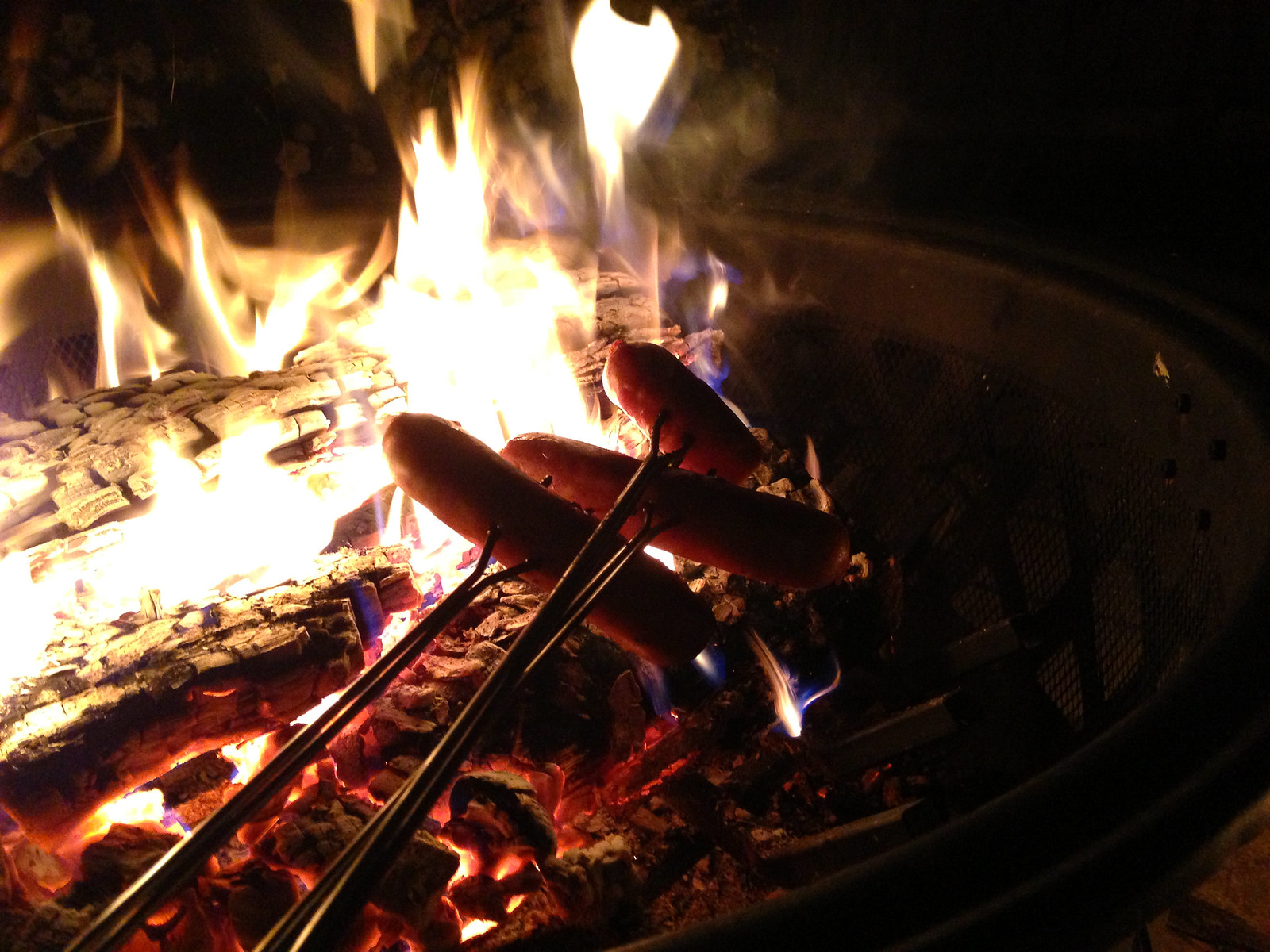In this nighttime image of an outdoor fire pit, we see a vibrant scene of glowing flames and smoldering logs. The fire pit itself is constructed from black metal, featuring a solid upper rim and a lower section of mesh that provides a view of the intense fire within. The bright yellow flames flicker upwards, illuminating the gray embers and charcoaled wood, with striking hues of orange, white, and hints of blue around the edges of the fire. 

In the center of the image, two long, silver metal forks are held over the fire, skewering three hot dogs. One fork holds two hot dogs, while the other holds one. The hot dogs appear to have been chopped in half, with their rounded ends facing left and the cut ends towards the bottom right. The flames cast a bright light on the scene, contrasting against the dark sky in the background, adding a warm, inviting glow to the moment of roasting hot dogs over the open fire.